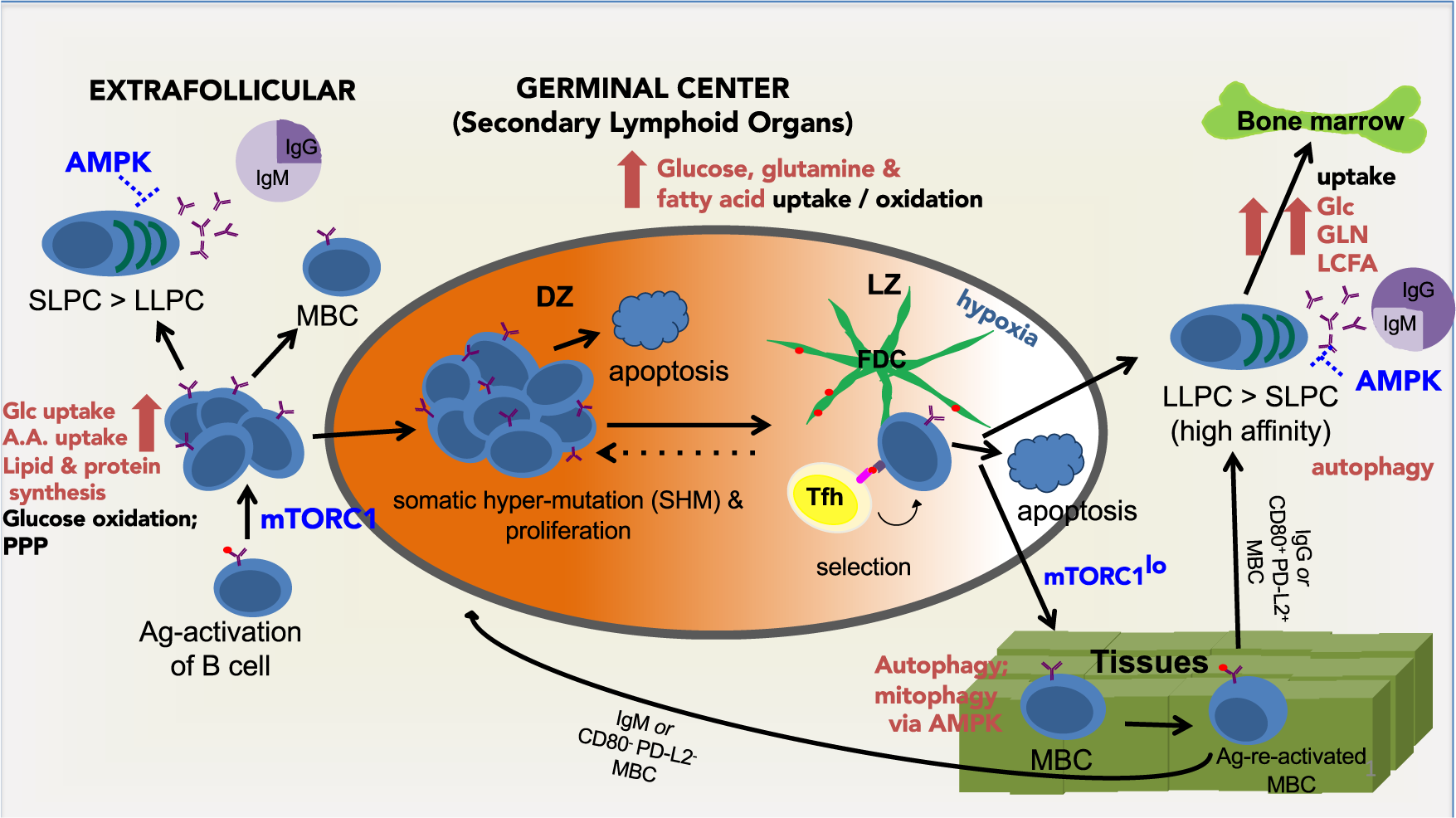This image is a digital scientific diagram in a landscape layout, with sides shorter than the top and bottom, and features a thin blue border at the top and right edges against a light off-white background. Centrally, it displays a wide oval with a gray border, transitioning from bright orange on the left to white on the right, containing numerous cell-like objects in blue, green, and yellow, each labeled with descriptions. Above the oval, a red arrow points upwards, labeled "Glucose, glutamine, and fatty acid uptake/oxidation," and situated above this is the title "GERMINAL CENTER," with the notation "Secondary lymphoid organs" in black.

Surrounding the central oval, the left section features several blue cell-like shapes, labeled "Extra follicular" in black text. To the right, a variety of illustrations include: blue circles with black text, a yellow circle labeled "TFH selection," and green lines converging like a spider web with additional cell-like objects and textual annotations in red, blue, and black. In the lower right, a green rectangle contains more blue circles and various colored texts, indicating different biological functions. At the upper right corner, a green bone illustration accompanied by blue and purple circles, red arrows, and more textual labels reflect locations depicted as "Bone marrow and tissues."

Overall, the diagram intricately illustrates cellular processes and environments within germinal centers, focusing on apoptosis, somatic hypermutation (HSM), proliferation, and hypoxia, clearly demarcating interactions among different cellular components and their functions through a combination of colored shapes, arrows, and labels.